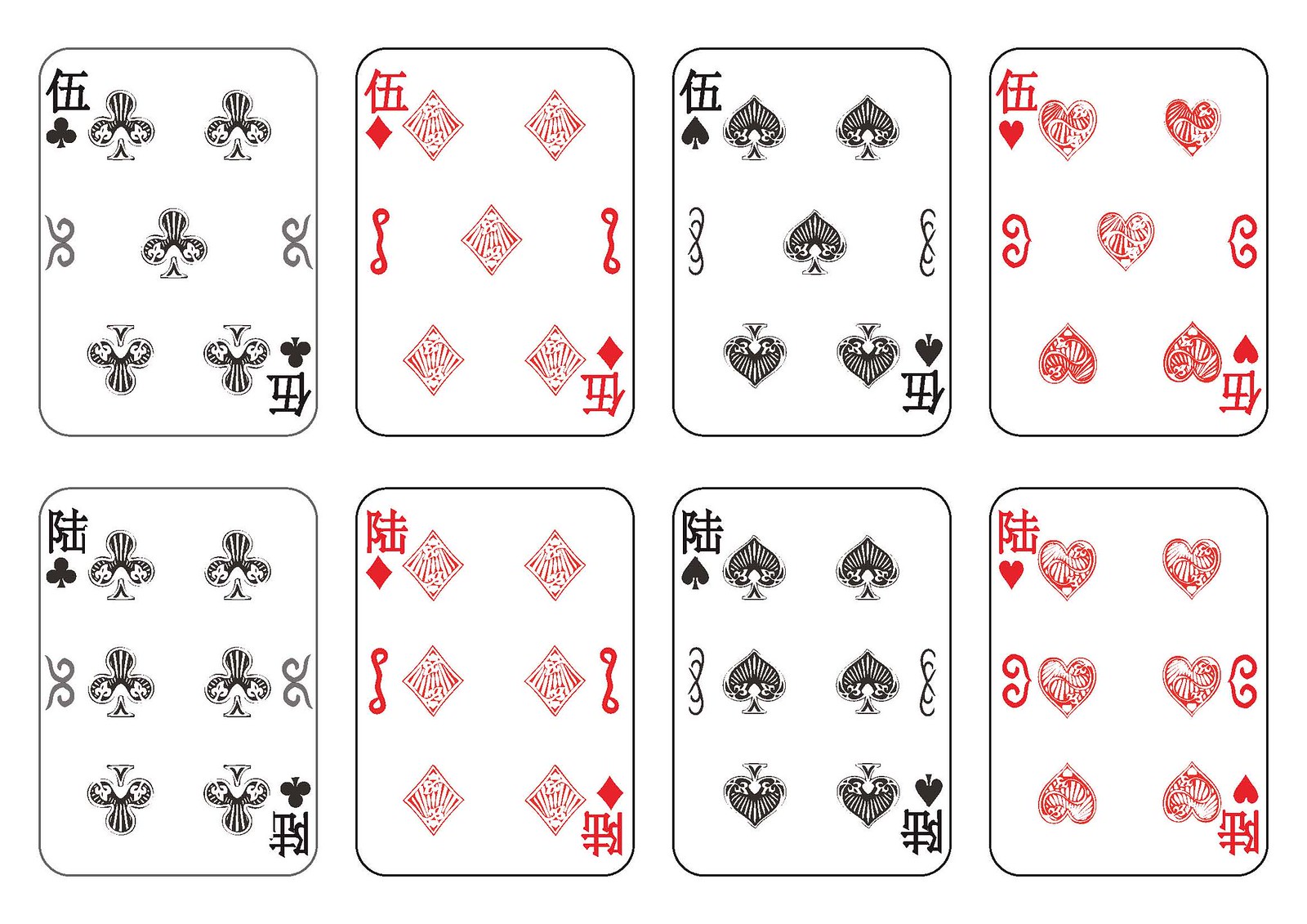The image features a set of eight playing cards arranged on a white background. Each card displays traditional Chinese characters, making it difficult to discern the numbers for those unfamiliar with the language. The cards are organized into two rows of four, with a pattern alternating between black and red. 

In the top row, from left to right, are: a black club, a red diamond, a black spade, and a red heart. In the bottom row, the sequence repeats with a black club, a red diamond, a black spade, and a red heart. 

Each card in the top row represents the number five, indicated by the respective number of suit symbols in the center of the cards. Similarly, the bottom row represents the number six. The suit symbols are drawn in intricate designs. The Chinese characters indicating the numbers are located at the top left and bottom right corners, similar to a standard Western playing card layout.